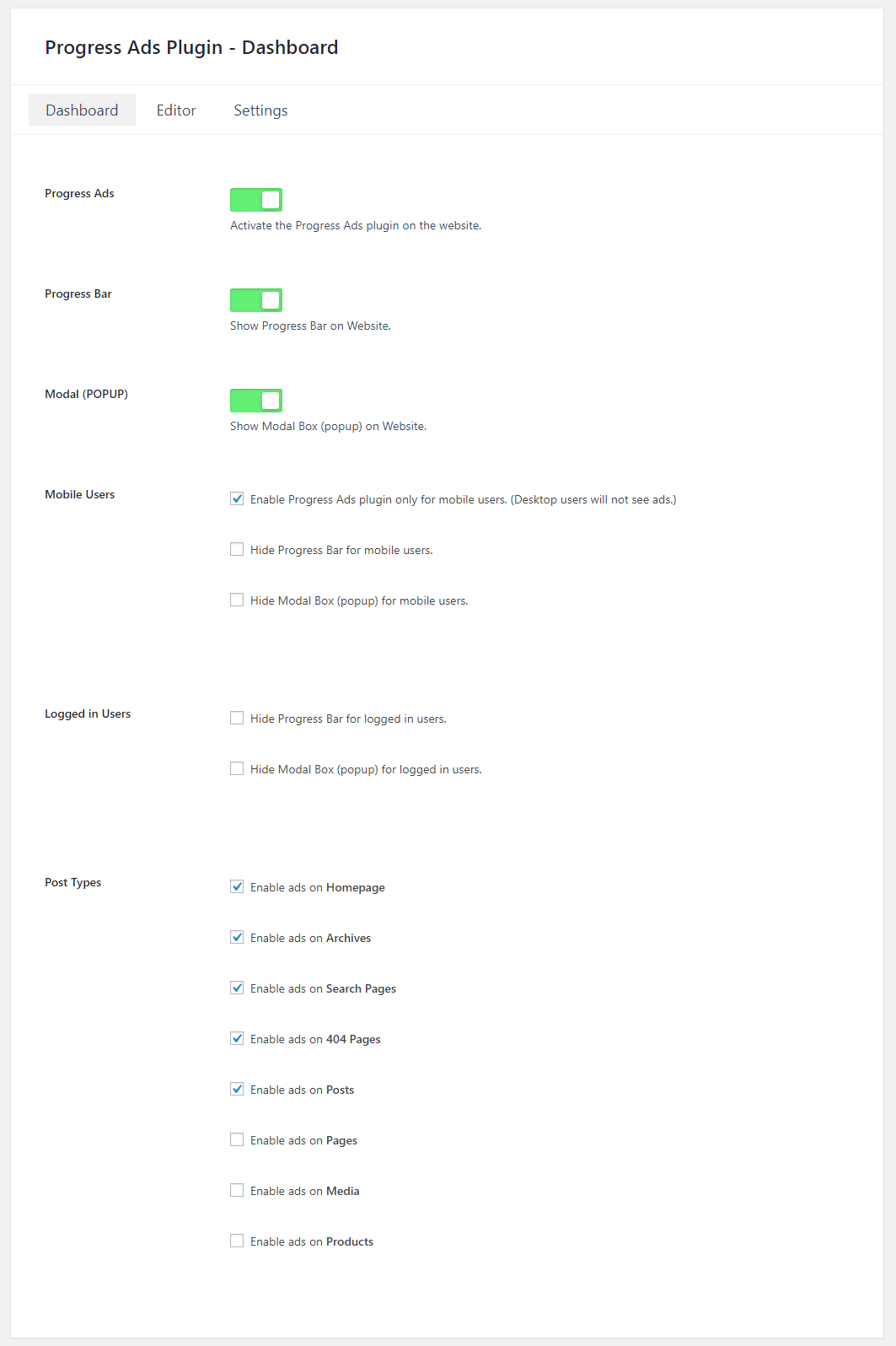The image showcases a user interface of a dashboard titled "Progress Ads Plugin, Dashboard." The primary navigation options include "Dashboard," "Editor," and "Settings," with "Dashboard" highlighted in gray, indicating it is the current view. 

The dashboard displays the status of various settings related to the "Progress Ads Plugin." The main settings are detailed as follows:

- **Progress Ads**: Enabled (indicated by a green checkmark), allowing the Progress Ads plugin on the website.
- **Progress Bar**: Enabled (indicated by a green checkmark), showing the Progress Bar on the website.
- **Modal Pop-up**: Enabled (indicated by a green checkmark), showing the Pop-up Box on the website.

Under the "Mobile Users" section, there are three configurable options, each with a checkbox:
1. **Enable Progress Ads Pop-ups only for mobile users** (checked),
2. **Hide the Progress Bar for mobile users** (unchecked),
3. **Hide the Modal Bar for mobile users** (unchecked).

The "Logged In" section has two choices for logged-in users, but neither is checked.

At the bottom of the interface, there is a "Post Types" section with eight available choices, of which the first five are checked. The enabled options appear to be:
1. Enable Progress Ads on the homepage,
2. Enable Progress Ads on the archive page,
3. Enable Progress Ads on the search page,
4. Enable Progress Ads on 404 error pages,
5. Enable Progress Ads on posts. 

This detailed configuration panel allows comprehensive control over where and how progress-related advertisements are displayed on the website.